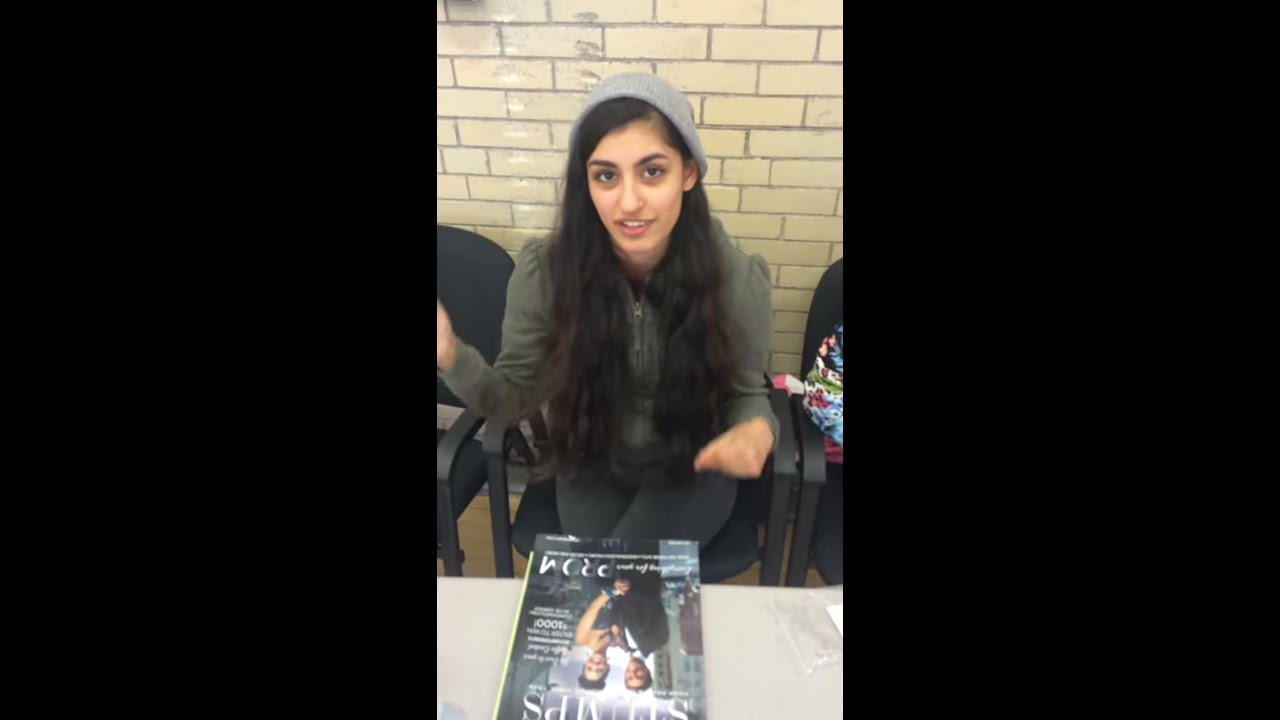In this color photograph, likely taken with a cell phone, we see a young woman with olive-colored skin and long dark hair, sitting directly in the center of the frame. She is wearing a dark gray zip-front top, a gray knit beanie cap, a green sweatshirt, and dark gray or black tights. The young woman has a grin on her face and looks directly at the camera, her hands outstretched in front of her, making a gesture. Behind her is a tan-colored brick wall, adding texture to the background.

She is seated on a linked, almost black chair, reminiscent of those found in a doctor's office, and has two empty chairs on either side of her. The chair to her left (the right side of the image) has someone partially cropped out, indicating there is another presence in the scene. 

In front of her is a white or beige table with a magazine laid flat on top of it, facing her. The magazine features a photograph of a man in a suit and a woman in formal attire holding hands and smiling. Also visible on the table to her right is a colorful cloth object, possibly a purse, featuring blues, pinks, whites, and greens. The overall setting could be an indoor or outdoor location, potentially a waiting area or an event where the woman is being interviewed or questioned by someone off-camera. The image is framed against a landscape background in black, emphasizing the central subject and her surroundings.